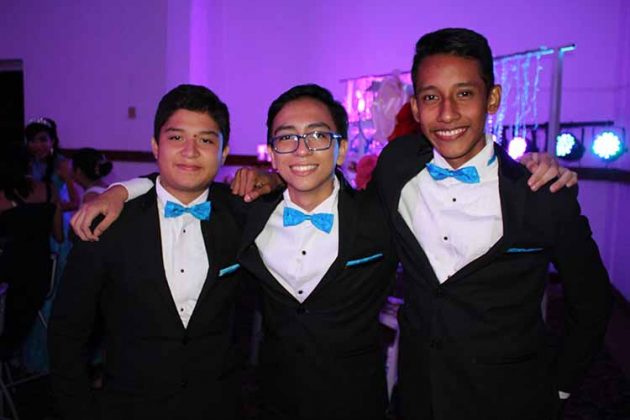This vibrant image captures three young boys, estimated to be between the ages of 12 and 15, smiling warmly for the camera at an event or party. They are standing in an atmospherically lit room, where purple-tinted lighting adds a festive glow against a predominantly white and black backdrop, enhanced by bright party lights and strings of lights on a banister to the right. Each boy is donned in a matching black suit with a crisp white tuxedo shirt, accessorized with a medium electric blue bowtie and a matching pocket square that provides a pop of vibrant color against their formal attire. The boy on the left, the shortest of the trio, sports thick brown hair and wears a subtle, closed smile. In the middle stands a boy with glasses and thinner brown hair, showcasing a broad grin with his teeth visible. The tallest boy on the right, with slightly darker skin and thick brown hair, also smiles broadly, his teeth visible as well. These boys, their arms affectionately wrapped around each other's shoulders, are the focal point of the photograph, capturing a moment of youthful camaraderie and joy.